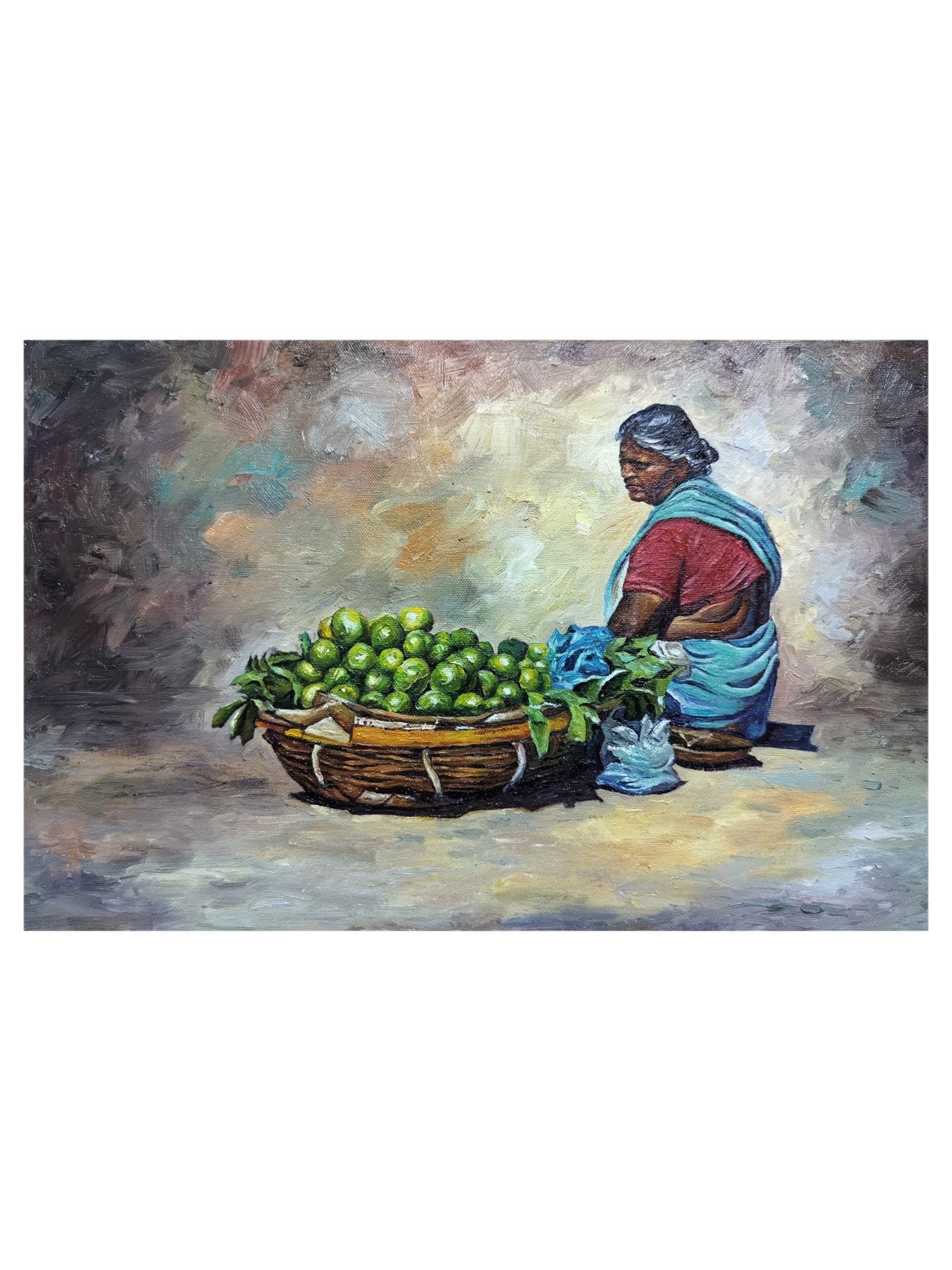A beautifully detailed painting depicts a middle-aged woman, possibly slightly older, seated on the ground. Her lower body is partially obscured by an abundant woven basket, overflowing with small green fruits or vegetables, accompanied by some leaves. The intricately woven basket serves as the focal point of the image, its contents piled high with vibrant green produce. Adjacent to the basket lies an indistinguishable object, possibly an open plastic bag or a piece of cloth.

The woman, positioned slightly to the right of the basket, gazes intently downward. She has dark hair interspersed with gray or white highlights and possesses dark skin. Her attire is reminiscent of traditional South Asian clothing, likely from India or Sri Lanka. She wears a short-sleeve shirt that reveals her midsection and is draped in blue cloth that wraps over her shoulder and around her waist. The background of the painting is an abstract blend of swirling colors, devoid of any distinct structures, enhancing the subject's prominence and creating a sense of timelessness.